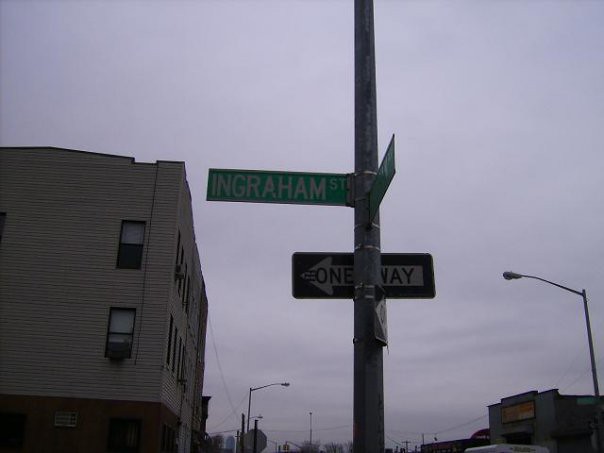In this high-quality photograph, the focal point is a silver metal pole prominently placed in the center of the image. Adorning the pole are several signs: two black signs with white arrows and "ONE WAY" written in black font, as well as a green sign with white lettering that reads "INGRAHAM STREET." Another green sign is partially visible, though its text is obscured. The background is bustling with urban elements, including light poles, power lines, and various businesses. One notable business features a light gray facade and an off-white sign. On the opposite side, a building with a mix of brick and light-colored siding is visible, showcasing several windows. Additional street signs are partially seen from the back, and in the far distance, stoplights can be faintly observed. The scene is set under an overcast, gloomy sky, adding a somber tone to the urban landscape.